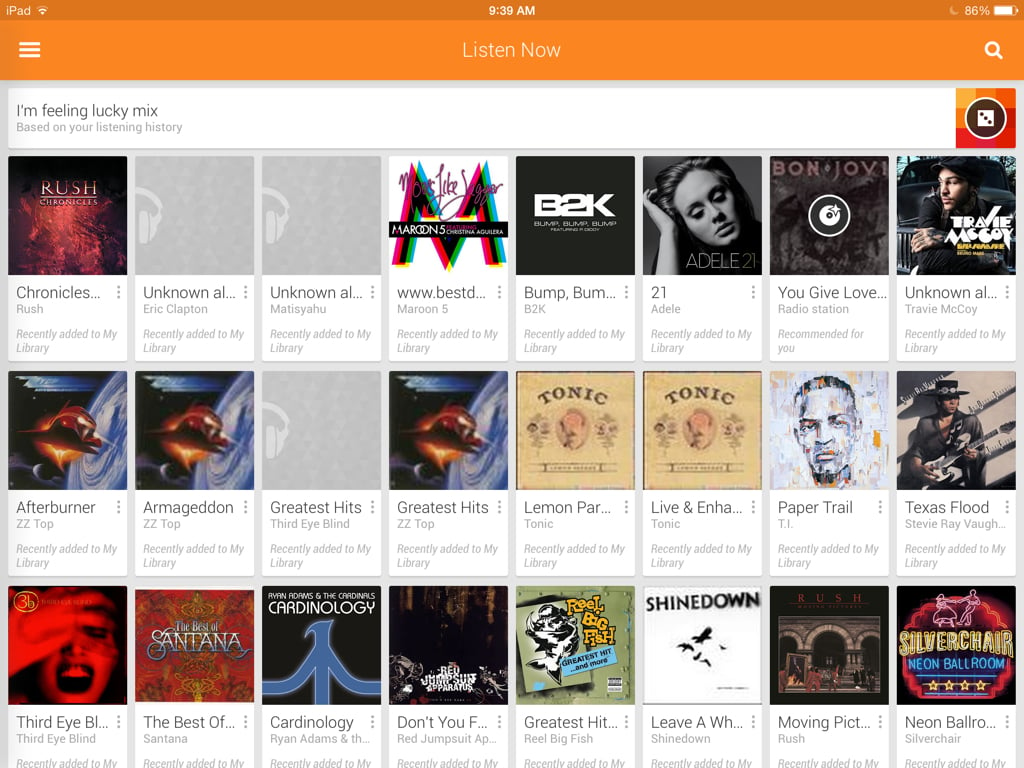This landscape-oriented screenshot appears to be taken from a music streaming application on an iPad. The screenshot shows a detailed interface filled with vibrant colors and various elements.

At the very top, there is a thin, dark orange status bar displaying an array of vital information. This includes the "iPad" label, the current time (9:39 AM), a greyed-out moon icon (likely indicating 'Do Not Disturb' mode), the Wi-Fi signal strength (missing the last bar), battery percentage (86%), and a horizontal battery icon with a white meter.

Below the status bar is an orange toolbar. On the left side, there is a white hamburger menu icon and next to it, the text "Listen Now" in white font. Adjacent to it, there is a white search bar, providing users with the option to look up their favorite tracks or artists.

Proceeding down the screen, a white horizontal bar stretches across the display with the title "I'm Feeling Lucky Mix based on your listening history" in black font. To the left of the text is an eye-catching image made up of different colored squares forming a large square. Centered within this square is a white circle with a black background featuring a white die showing the number 3 in black dots.

Below this, the user’s music recommendations are laid out in a grid format consisting of 3 rows and approximately 9 columns, showcasing an impressive variety of songs. Artists featured in this selection include notable names such as Rush, Eric Clapton, Maroon 5, Adele, Travie McCoy, ZZ Top, Third Eye Blind, Tonic, T.I., Stevie Ray Vaughan, Santana, Ryan Adams, The Red Jumpsuit Apparatus, Reel Big Fish, and Rush again, indicating a diverse and eclectic taste in music.